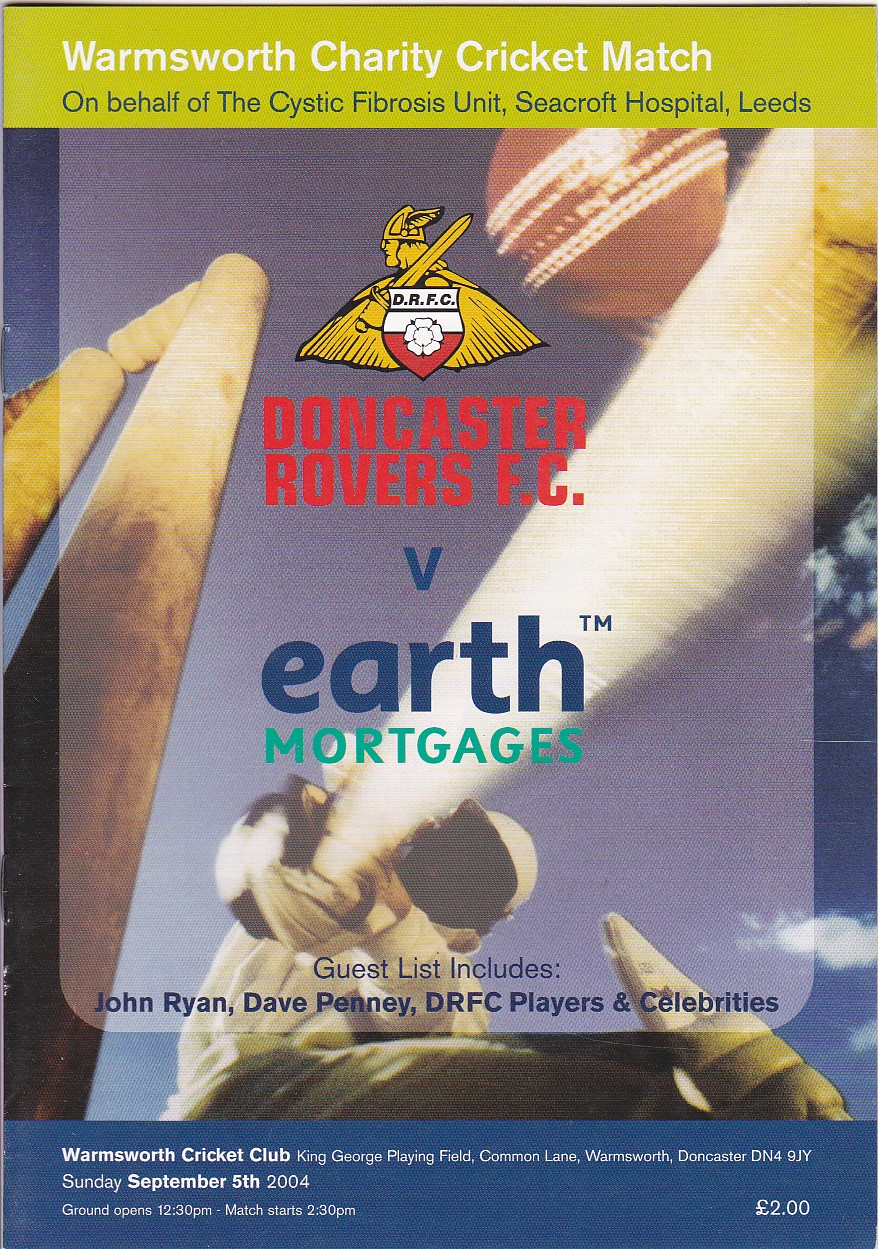The image is a detailed poster advertising the Warm S'more Charity Cricket Match on behalf of the Cystic Fibrosis Unit at Seacroft Hospital in Leeds. The poster includes a prominent logo featuring a man with wings holding a sword. The primary event features the Doncaster Rovers FC competing against Earth Vortices. It details that special guests include John Ryan, Dave Penny, DRFC players, and various celebrities. The central part of the poster showcases an action shot of a cricketer mid-swing, bat blurred for emphasis, with the person positioned center and angled upwards. It also lists event details: taking place at Wormsworth's Cricket Club, King George Playing Field, Common Lane, Wormsworth, Doncaster, DN4 9JY, on Sunday, September 5th, 2004. The ground opens at 12:30 PM, and the match starts at 2:30 PM, with an entry price of £2.